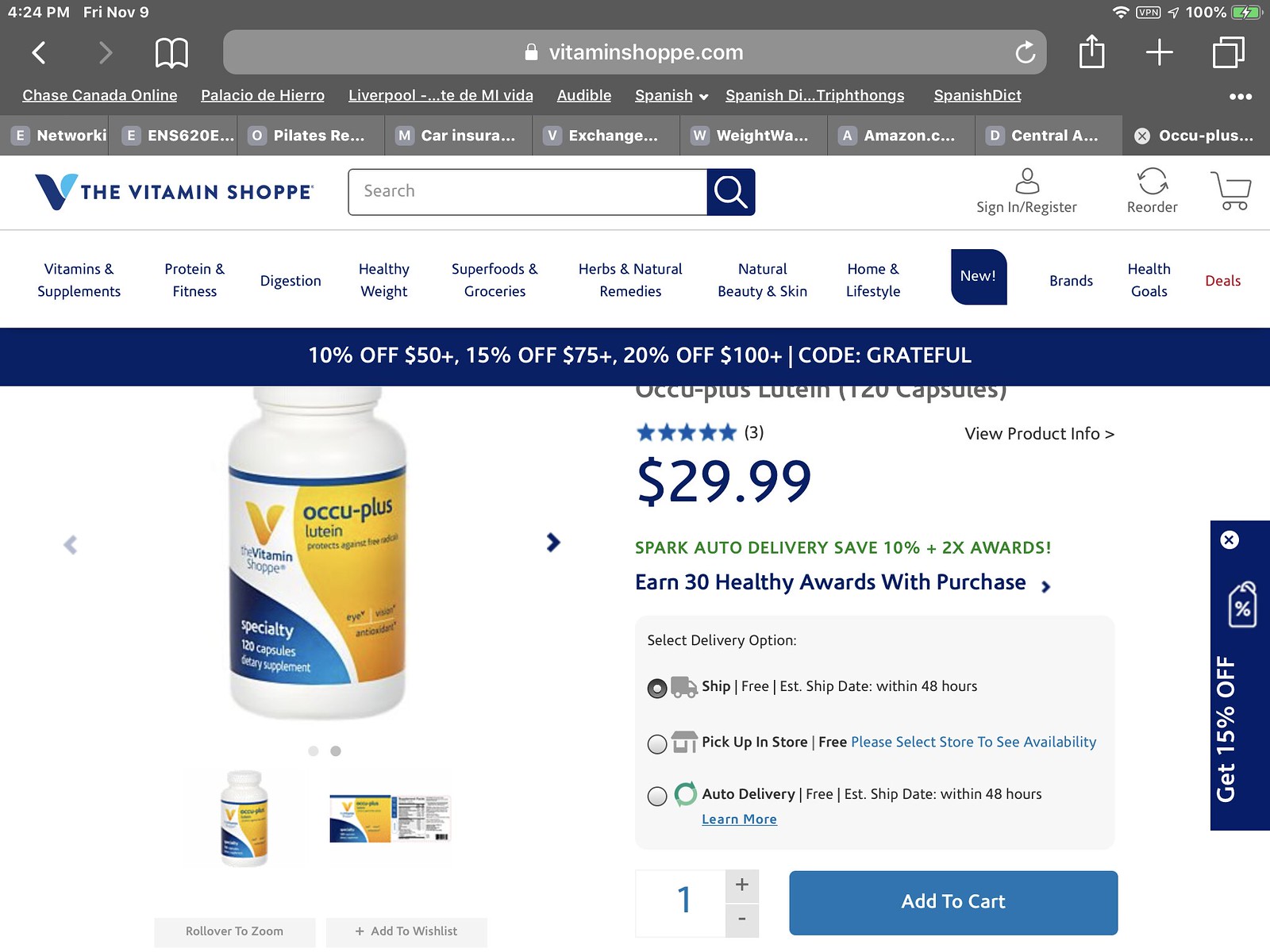This is a detailed screenshot of a webpage from Vitaminshop.com taken from an Apple device, likely an iPad, as evidenced by the icons in the upper right corner. At the top left, the website URL is secured with a lock symbol. Several tabs are open, including Chase Canada Online, Palacio de Hierro, Liverpool, Audible, and various Spanish language resources.

The main focus of the page is a product named Occuplus Lutein Specialty, a dietary supplement designed for eye health and antioxidant protection. The white bottle has a blue and yellow label, contains 120 capsules, and is priced at $29.99. It has a five-star rating based on three customer reviews. 

A promotional banner offers discounts with a coupon code "GRATEFUL": 10% off orders over $50, 15% off orders over $75, and 20% off orders over $100. Additionally, there's an option to "Spark Auto Delivery" to save 10% and earn double rewards. The banner also indicates that purchasing this item would earn 30 healthy award points.

The website’s navigation includes categories such as Vitamins and Supplements, Protein and Fitness, Digestion, Healthy Weight, Superfoods and Groceries, Herbs and Natural Remedies, Natural Beauty and Skin, Home and Lifestyle, New Brands, Health Goals, and Deals.